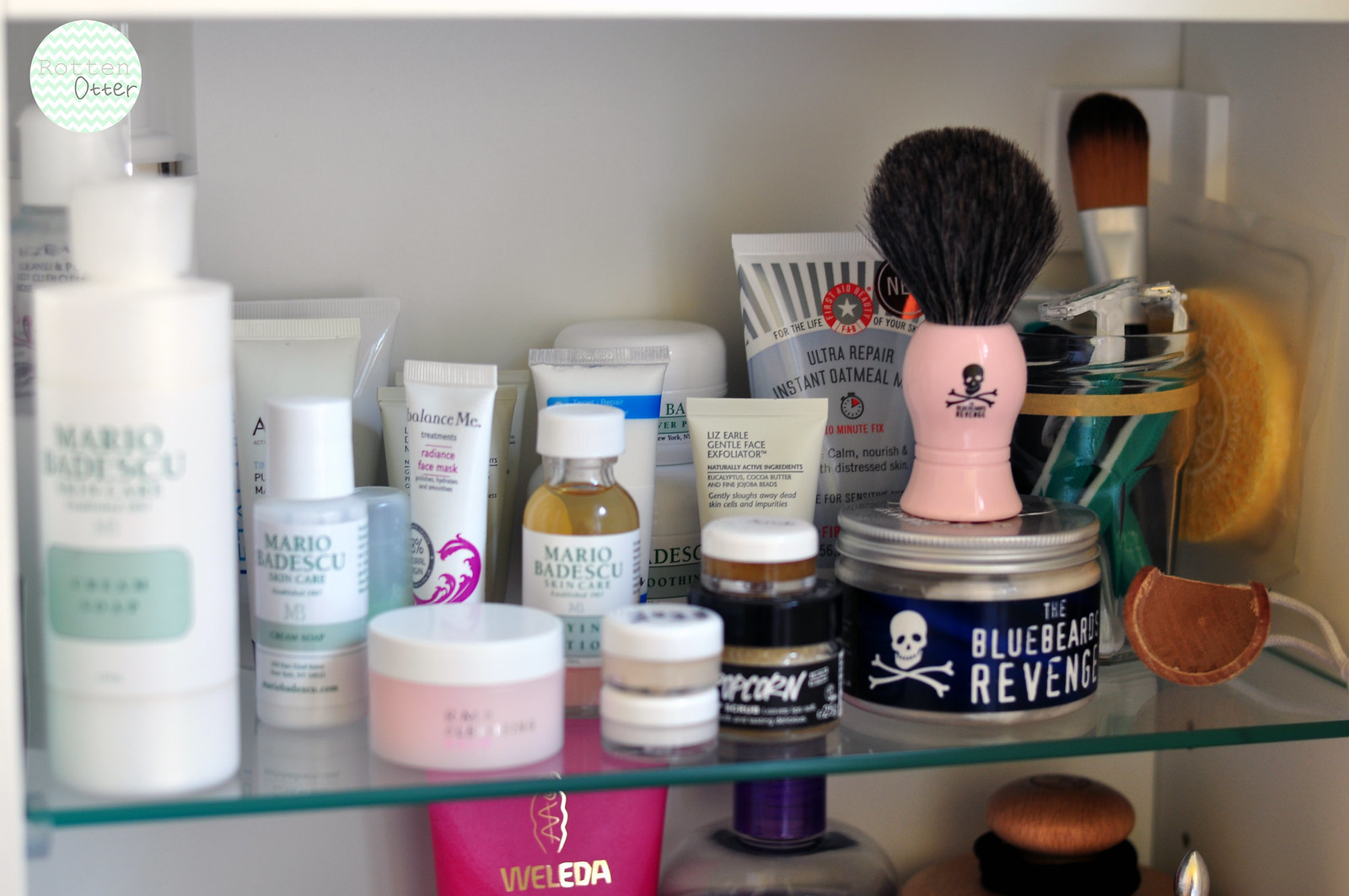The photograph captures the interior of a well-organized medicine cabinet, showcasing a variety of personal care products arranged meticulously on a glass shelf. 

On the lower shelf, starting from the left, there's a pink bottle with the brand name "Welita" accented in gold print. Next to it are two other unidentified bottles. 

The upper glass shelf is populated with several items: beginning from the left, there's a white bottle with a white cap labeled "Mario." Adjacent to this is a smaller bottle also from the Mario Badescu brand. Next to it, we see a small tub with a white cap and pink container, with another Mario Badescu product situated behind it. Moving further right, there's a clear glass bottle with a black top and label, partially displaying the word "Popcorn." Continuing rightward, there's another tub with a silver top and a label featuring a skull and crossbones, reading "The Bluebeards Revenge," which might be a hair gel. Resting atop this tub is a kabuki-style brush, possibly used for applying shaving cream or makeup. 

Behind these items, a plastic container labeled "Ultra Repair Instant Oatmeal," likely a skin product, is visible. 

In the upper right corner of the cabinet, two upright disposable razors and a makeup brush, suitable for applying concealer, are placed in a glass. Additionally, there is a small, thin orange sponge made of loofah-like material.